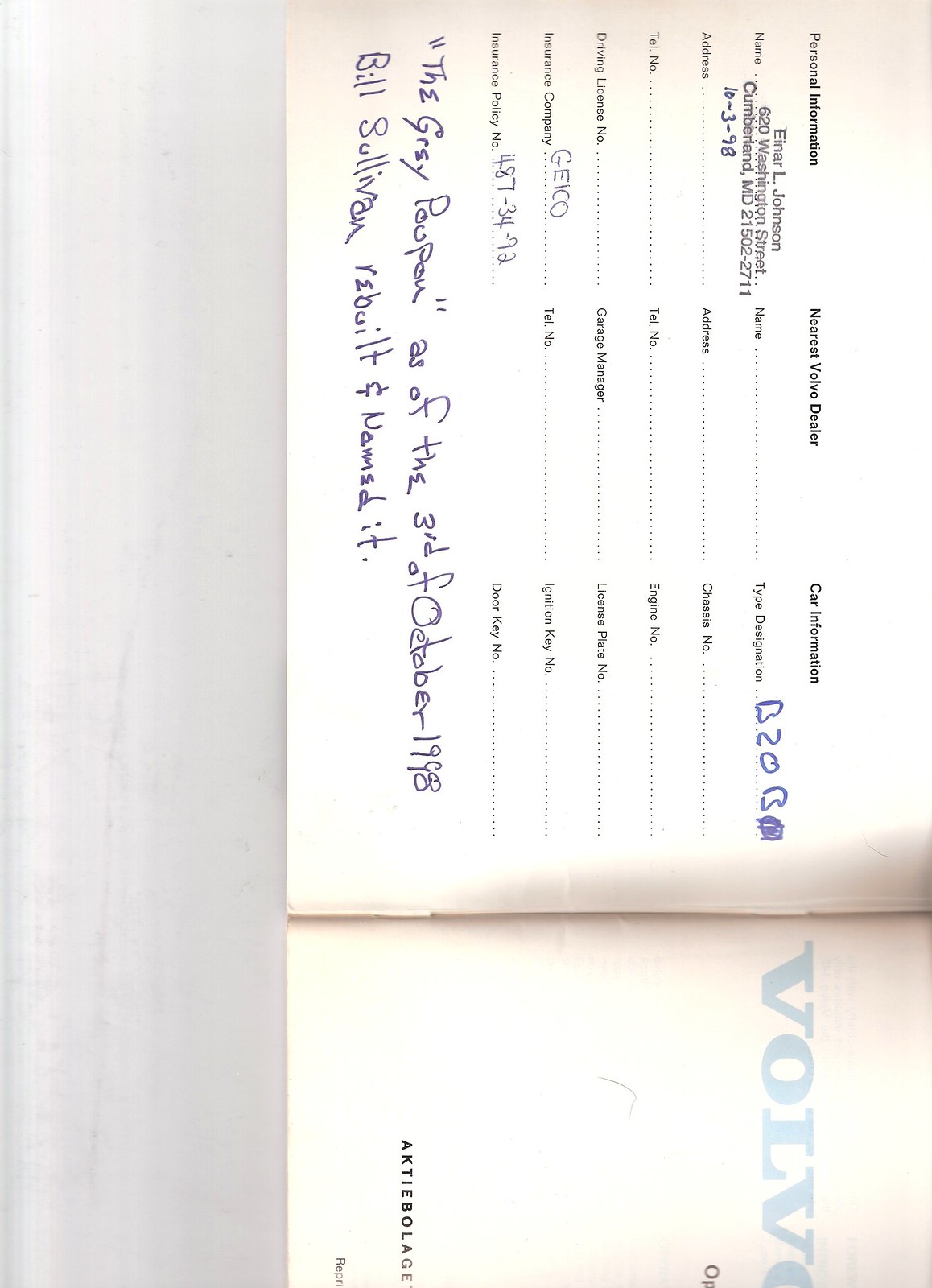The image shows a scanned, slightly rotated image of a Volvo manual or warranty booklet placed on a white sheet of paper or possibly a desk. The booklet appears to be open, displaying a form that records personal and car information. The form is partially filled out with detailed entries. Under the personal information column, the name listed is Einar L. Johnson, residing at 620 Washington Street, Cumberland, Maryland, 21502-2711, dated October 3, 1998. Information about the nearest Volvo dealer is left blank. The car information section includes the type designation B20B. The insurance company is noted as GEICO with policy number 487-3492. Notably, the bottom of the form has a handwritten note stating, "The Grey Poupou, as of the 3rd of October, 1998, Bill Sullivan rebuilt and named it." On the right half of the booklet, stapled together, the Volvo name and logo in blue are visible, pointing towards it being an official and possibly older document.